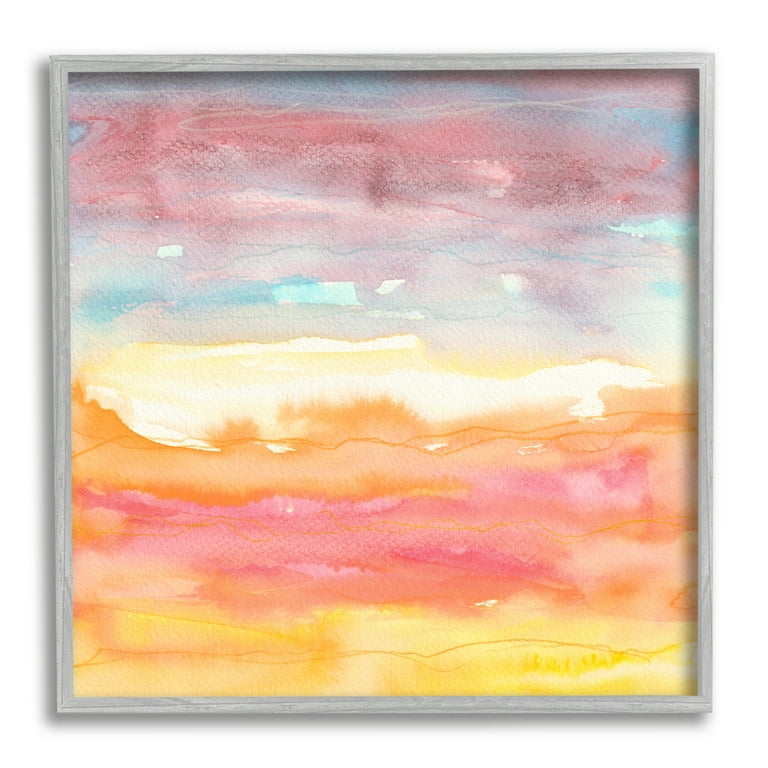This is a detailed photograph of an abstract watercolor painting characterized by multiple layers of colors that seamlessly blend into each other. The image is square and features a light gray frame with a shadow cast along the left and bottom edges, all set against a white background. From top to bottom, the painting transitions through a textured spectrum of hues: it starts with a greenish-gray and flows into pink, then light blue. This segment transitions into a subtle yellow, followed by white, and then a distinct orange. Below the orange layer, the colors shift into pink which eventually deepens into red. Finally, the composition culminates in a solid yellow layer at the bottom, which has an orange line running down its center. The colors smear and blur together, creating an uninterrupted gradient from darker and cooler tones at the top to warmer and lighter tones at the bottom. The painting is devoid of any specific subjects, focusing purely on the interplay of colors and textures.